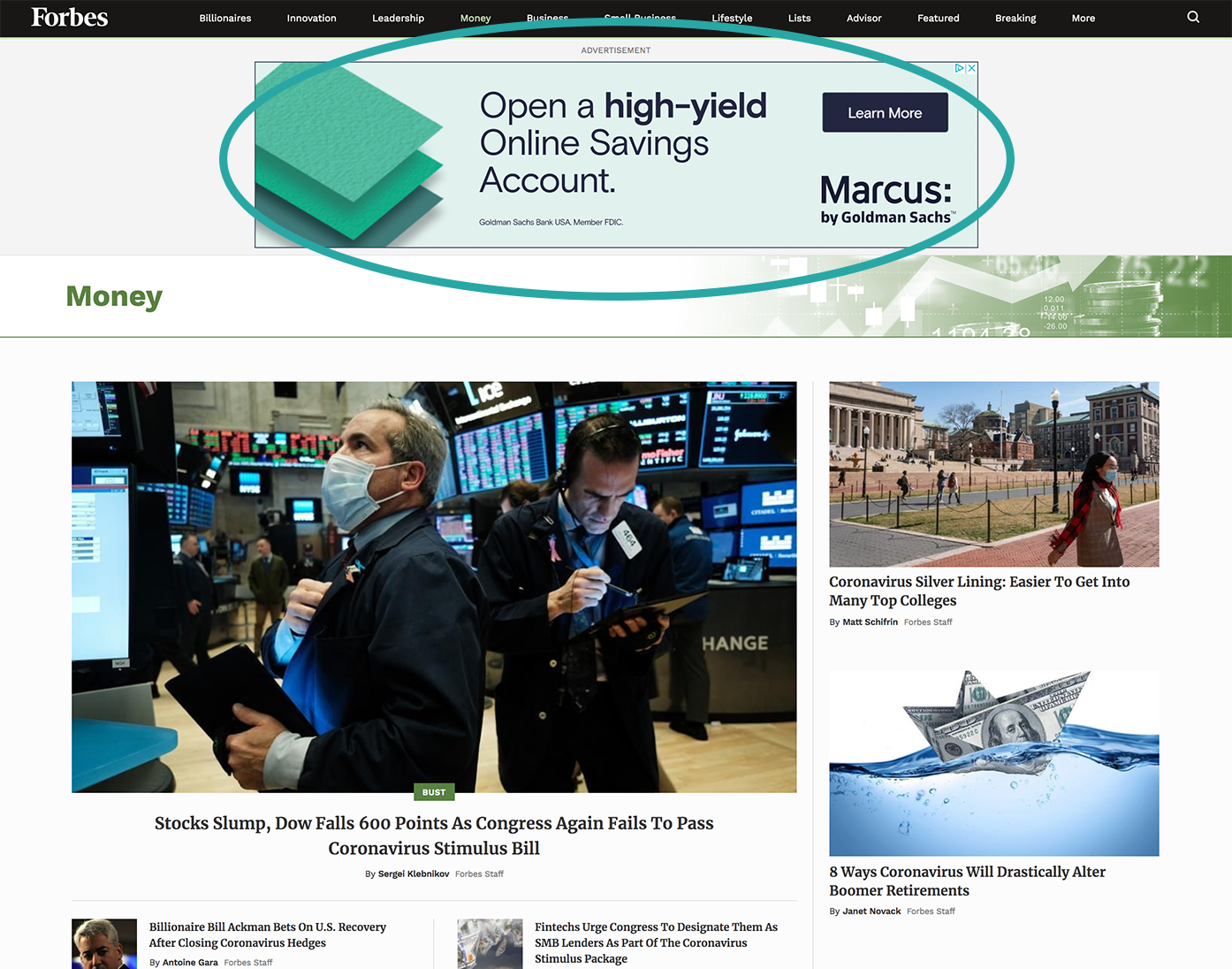This image is a screenshot of the Forbes website homepage. At the top of the screen, the Forbes logo is prominently displayed in the top-left corner. Adjacent to the logo, a horizontal navigation bar features various sections including Billionaires, Innovation, Leadership, Money, Business, Small Business, Lifestyle, Lists, Advisor, and Breaking. The last visible menu item is partially obscured, possibly indicating "Small Business." On the far right of this navigation bar is a search icon for website queries.

Beneath the navigation bar, there is a conspicuous advertisement by Goldman Sachs promoting a high-yield online savings account, highlighted by a green oval drawn around it. 

Below the advertisement, the content section of the Money category is currently displayed. This section features articles accompanied by images. One of the highlighted stories reports on a sharp decline in stock prices, titled "Stock Slump: Dow Falls 600 Points as Congress Again Fails to Pass Coronavirus Stimulus Bill." Another article features billionaire Bill Ackman and his optimistic bets on the U.S. economy's recovery after closing his coronavirus hedge positions. Additional articles and images populate this section, providing further financial news and updates.